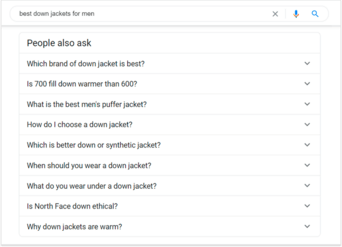This image is a cutout from the middle of a SERP (Search Engine Results Page) that specifically highlights the "People Also Ask" section. At the top, the search query "Best Down Jackets for Men" is prominently displayed in the query box. Below this, the "People Also Ask" section is visible, containing a list of nine expandable questions related to down jackets. These questions, in order, are:

1. Which brand of down jacket is best?
2. Is 700 fill down warmer than 600?
3. What is the best men's puffer jacket?
4. How do I choose a down jacket?
5. Which is better, a down or synthetic jacket?
6. When should you wear a down jacket?
7. What do you wear under a down jacket?
8. Is North Face down ethical?
9. Why are down jackets warm?

This section aims to provide users with related inquiries and quick-access answers to enhance their search experience. In the context of a full SERP, additional elements such as advertisements and more detailed guides or product selections would be visible both above and below this snippet. If you were researching the best down jackets for men, this "People Also Ask" section provides a concise set of frequently asked questions that could help guide your purchasing decision.